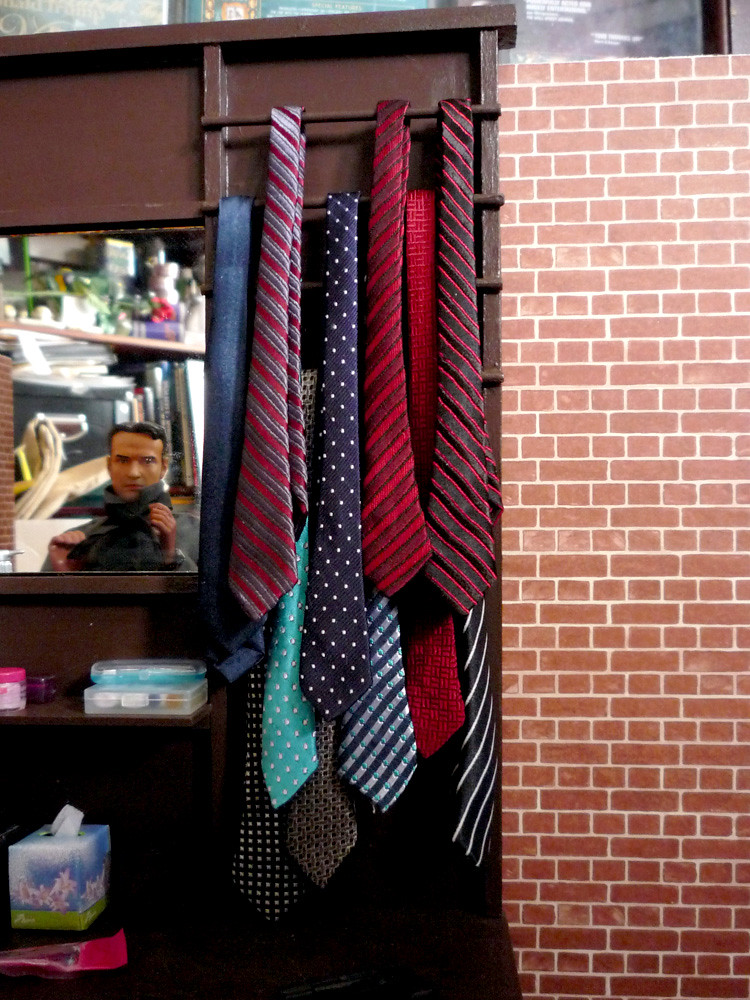This image depicts a highly detailed diorama resembling a miniature room. A prominent feature is a wooden tie rack against a red brick wall, displaying around 10 to 12 men's ties in an array of designs including stripes and polka dots, in colors like reds, blues, and grays. Adjacent to the tie rack, there is a wooden shelving system which accommodates various tiny items, including a box of tissues and transparent containers with small objects. To the left, a reflective surface, likely a mirror, shows the image of a lifelike figurine of a man with short dark hair, wearing a scarf. The detailed craftsmanship and realistic features of the scene, from the texture of the brick wall to the miniature accessories, suggest that this is a dollhouse diorama, showcasing an impressive array of doll-sized, yet incredibly lifelike, items.